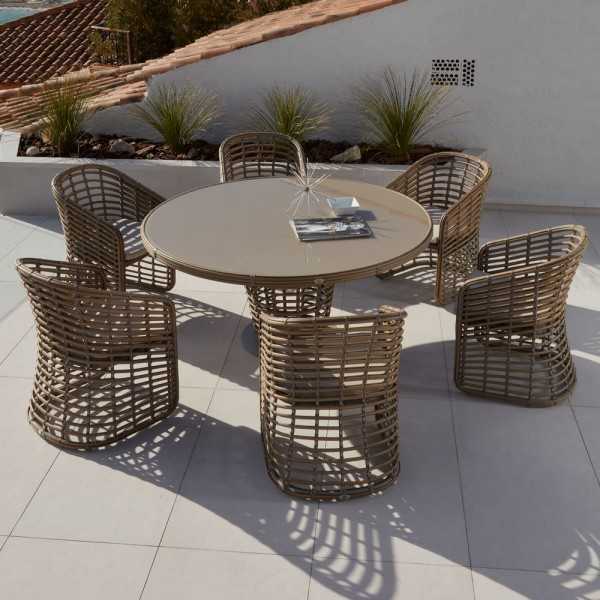This outdoor photograph, taken on a bright sunny day, captures a patio area that appears to be on the penthouse level of a building. The scene features a paved floor with rectangular cement tiles. Central to the composition is a wicker patio set, consisting of a round wicker table with a dark beige top and a wicker base, surrounded by six matching wicker chairs, each adorned with a small seat cushion. On the table, a star-shaped decorative centerpiece catches the eye, alongside a magazine and a small white bowl, possibly an ashtray or dipping dish. In the background, orange roofing and a planter with four plants are visible, adding layers of texture and color to the setting. The predominant colors in the photograph are shades of brown, white, green, and black, interspersed with lighter brown hues. Shadows from the sunlight add depth to the image, highlighting the fine details of the woven wicker furniture.